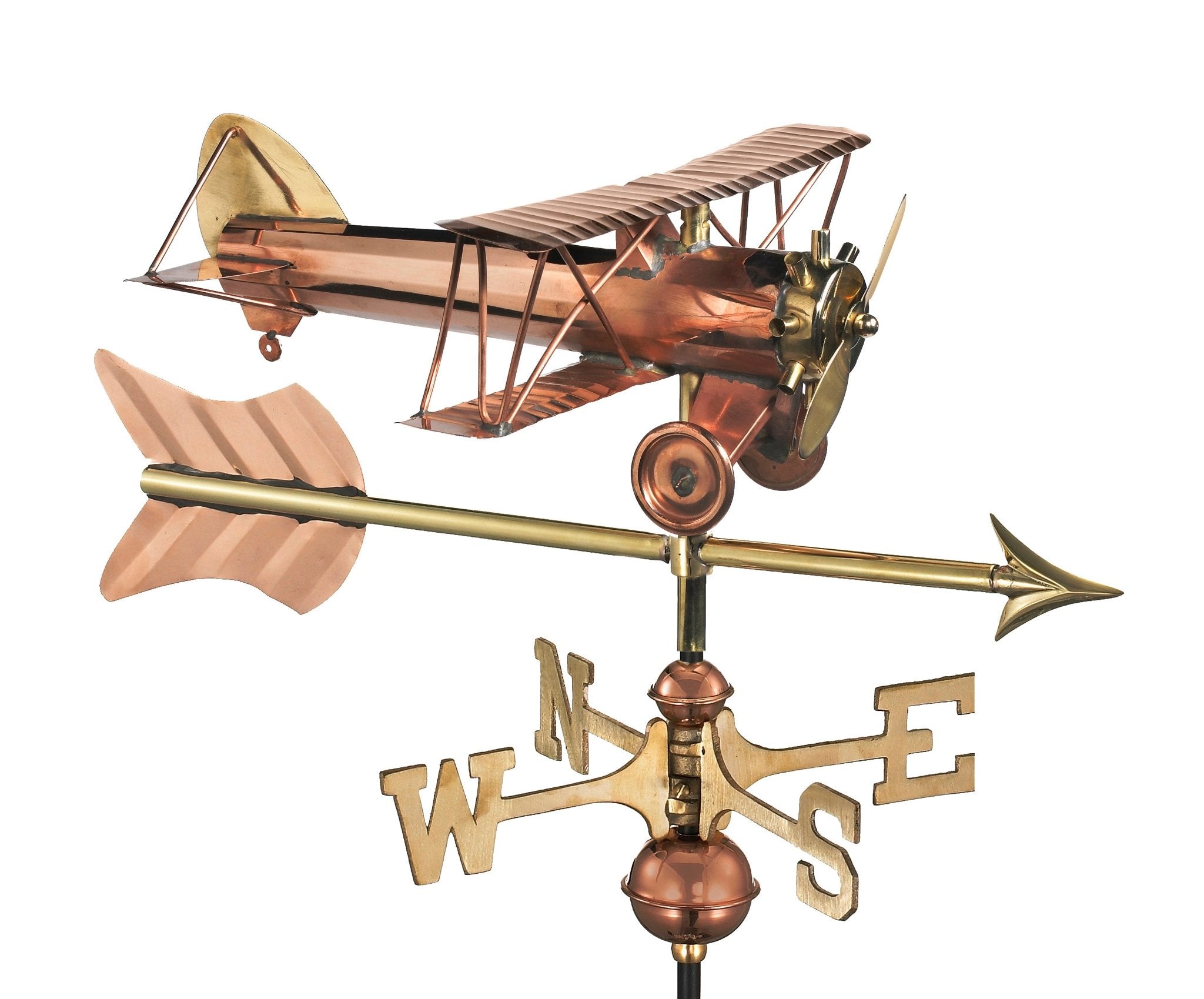The image is a detailed, full-color photograph of a metal weather vane, displayed against a plain white background typical of a stock image. The main vertical pole supports four rods extending outwards, labeled with the cardinal directions: N, S, E, and W, indicating north, south, east, and west. These rods are likely made of brass or copper, matching the metallic theme of the entire structure. Above these directional indicators is a finely detailed arrow, also metallic, presumably brass or copper, pointing to the right. Atop the arrow sits a meticulously crafted model of a biplane, featuring two sets of wings, a propeller at the front, and wheels, all rendered in the same brass or copper coloration. The weather vane includes several spherical elements along the main pole, adding to its ornate design. This image, devoid of any background distractions, focuses entirely on highlighting the intricate details and craftsmanship of the weather vane.